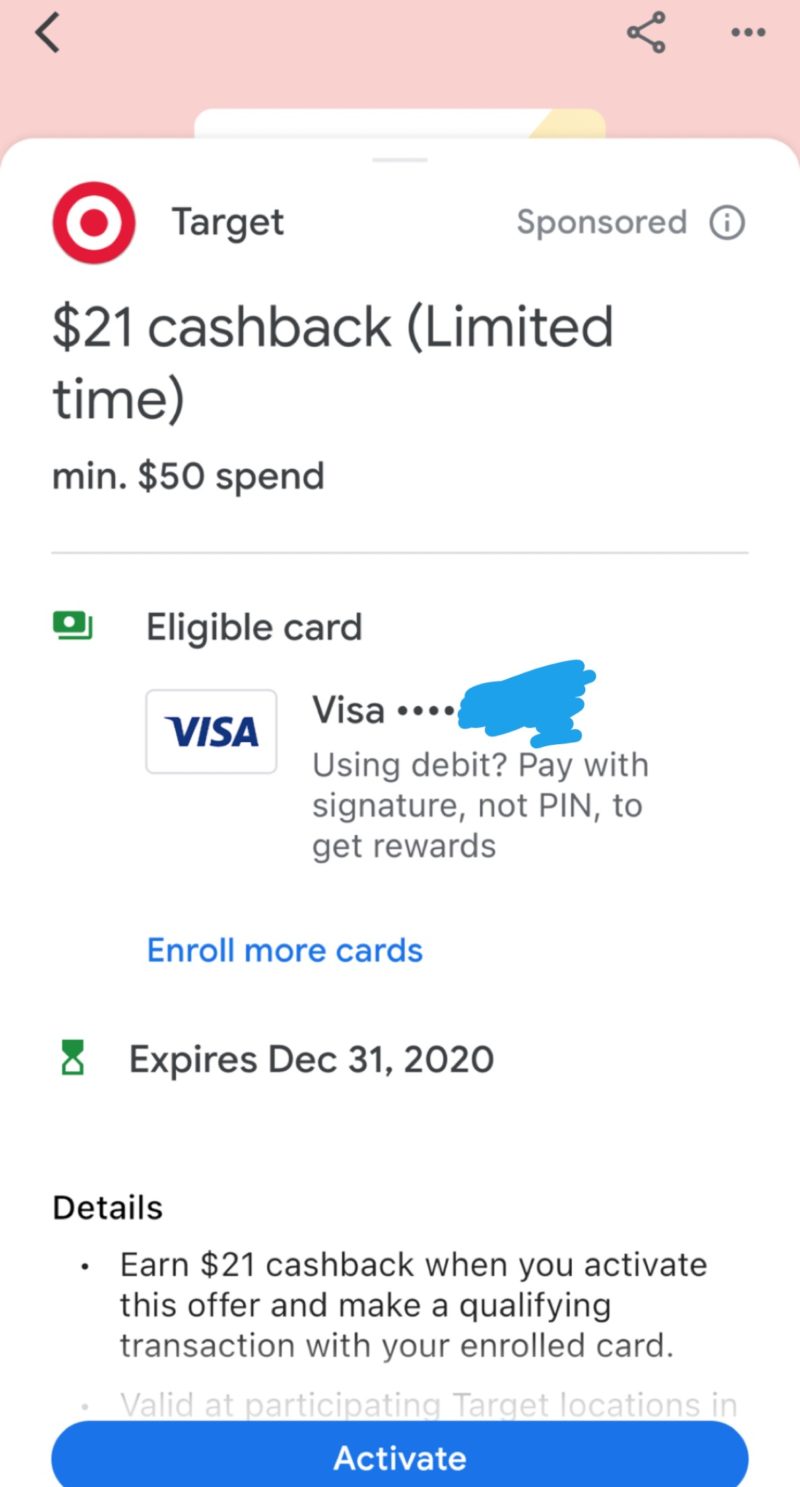A smartphone screen displays a partially scrolled-down Target webpage with a predominantly pink header, which includes three dots, an arrow, and a connective graphic consisting of an arrow with four black spheres at each end. Overlayed on this page is a promotion for a limited-time offer: "$21 cash back" with a minimum purchase of $50. The text "sponsored" is displayed next to Target's red bullseye logo.

At the top of the promotion, encircled in gray, is an eye icon, indicating additional information. Below this, the details are written in clear black font. The offer specifies eligibility criteria and outlines the steps needed to earn cashback. A green icon signifying a currently linked eligible card is visible, followed by a partially obscured Visa logo, marked out in blue ink. Instructions emphasize using a debit card with a signature, not a PIN, to qualify for the reward.

Further details include a link to "enroll more cards" in blue text and an expiration date of December 31st, 2020, accompanied by a green hourglass icon. The page also has an actionable "Activate" button in solid blue at the bottom, encouraging users to engage with the offer.